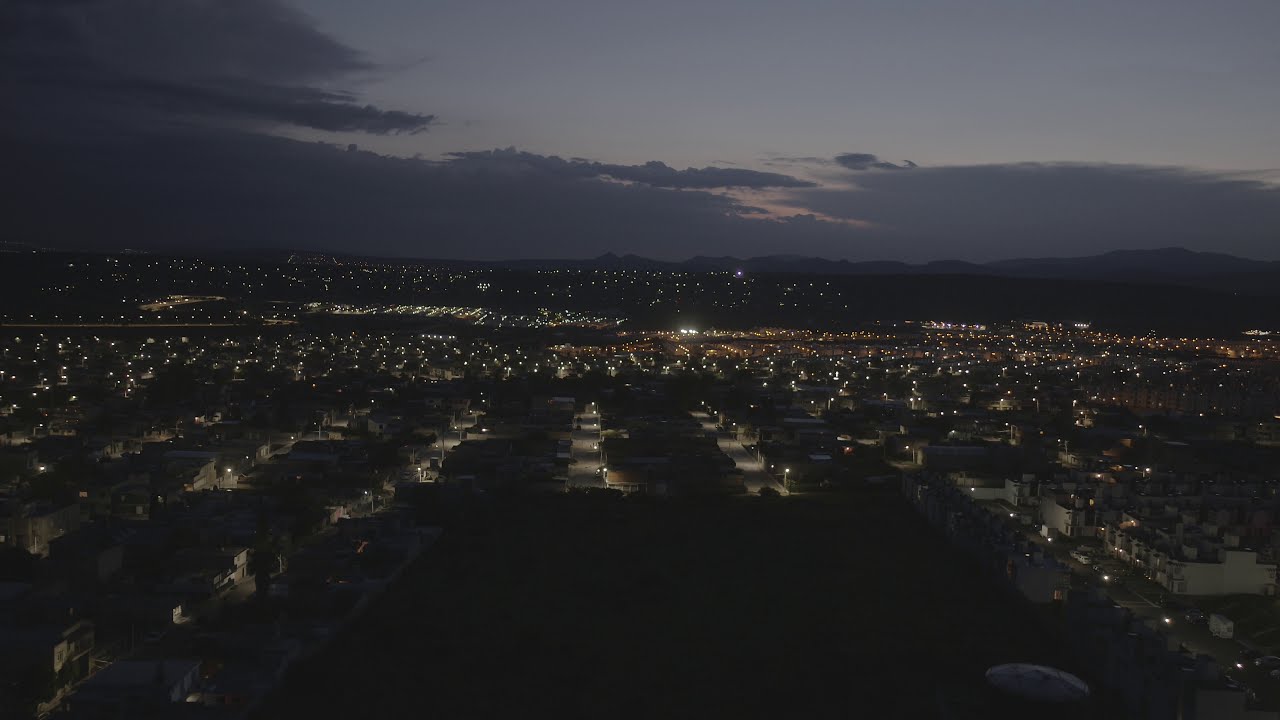In this elevated nighttime cityscape view taken approximately 100 feet above the ground, the scene is primarily characterized by its flat expanse, intermittently dotted with lights from buildings and streetlights. The camera is directed straight ahead, capturing a horizon with shallow hills on the right side. The sky above retains a hint of twilight blue and orange from a nearly set sun, while clouds drift out from the horizon and the left edge of the frame. The ground below is predominantly dark, with the foreground, particularly in the bottom middle, completely enveloped in blackness. The city is sparsely illuminated, with lights highlighting the scattered buildings and streets, giving a faint outline of the town's structure amidst the enveloping darkness.